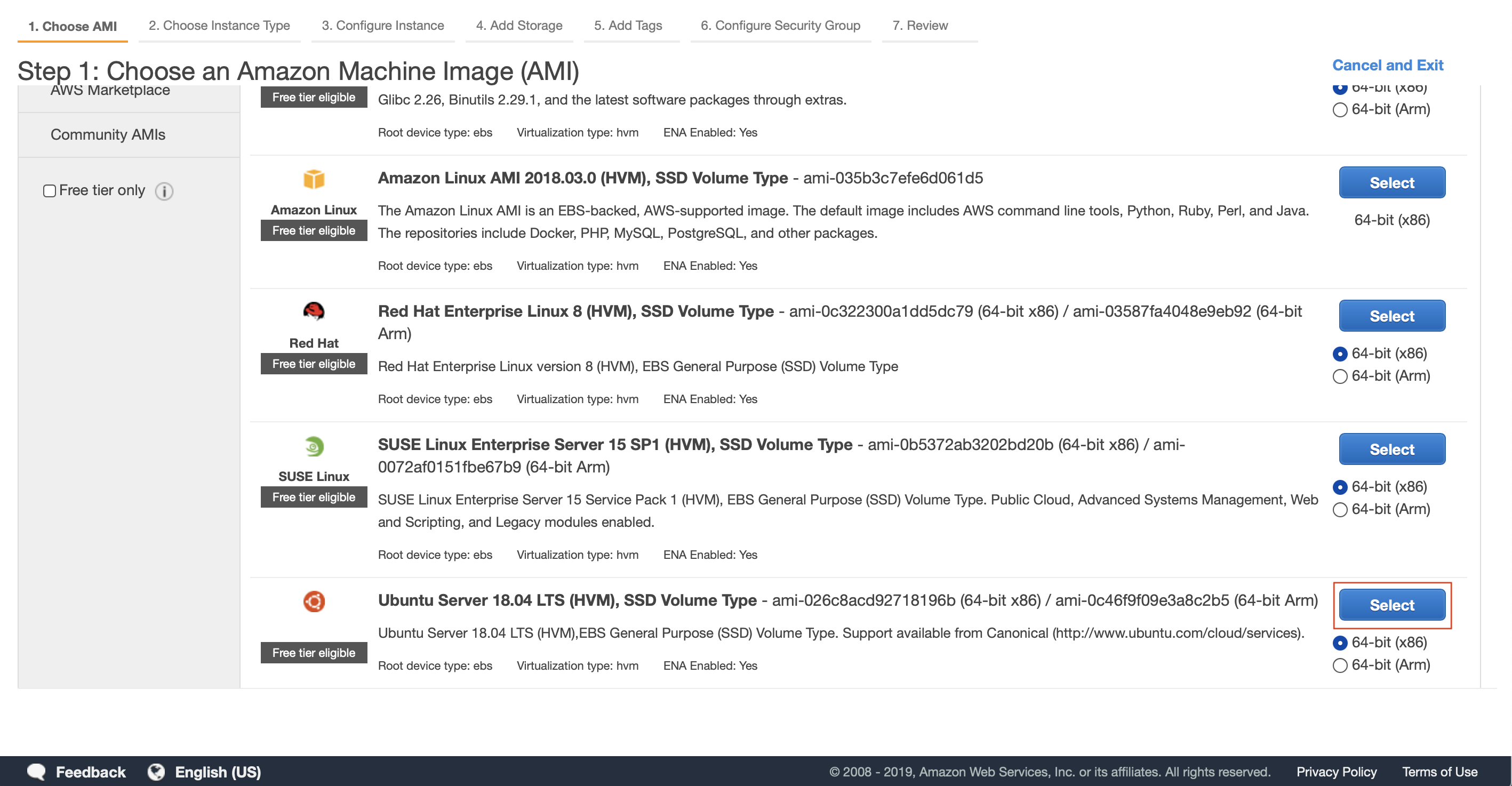**Detailed Caption:**

In the image, four selectable Amazon Machine Images (AMIs) are presented on a user interface for configuring a new instance on Amazon Web Services (AWS). The options listed include:

1. **Amazon Linux AMI 2018** - HVM, SSD volume type
2. **Red Hat Enterprise Linux 8** - HVM, SSD volume type
3. **SUSE Linux Enterprise Server 15 SP1** - HVM, SSD volume type
4. **Ubuntu Server 18.04 LTS** - HVM, SSD volume type

Each image is available in both 64-bit x86 and 64-bit ARM architectures, as indicated by the respective selection options beside each AMI. The "Select" button for each image is accompanied by these architecture choices, and the specific "Select" button for the Amazon Linux AMI 2018 is visually highlighted with an orange border, indicating it's currently chosen. On the right side of the interface, there are options to "Cancel" and "Exit" the selection process. The clarity in details ensures users can identify and select the appropriate AMI and architecture for their needs.